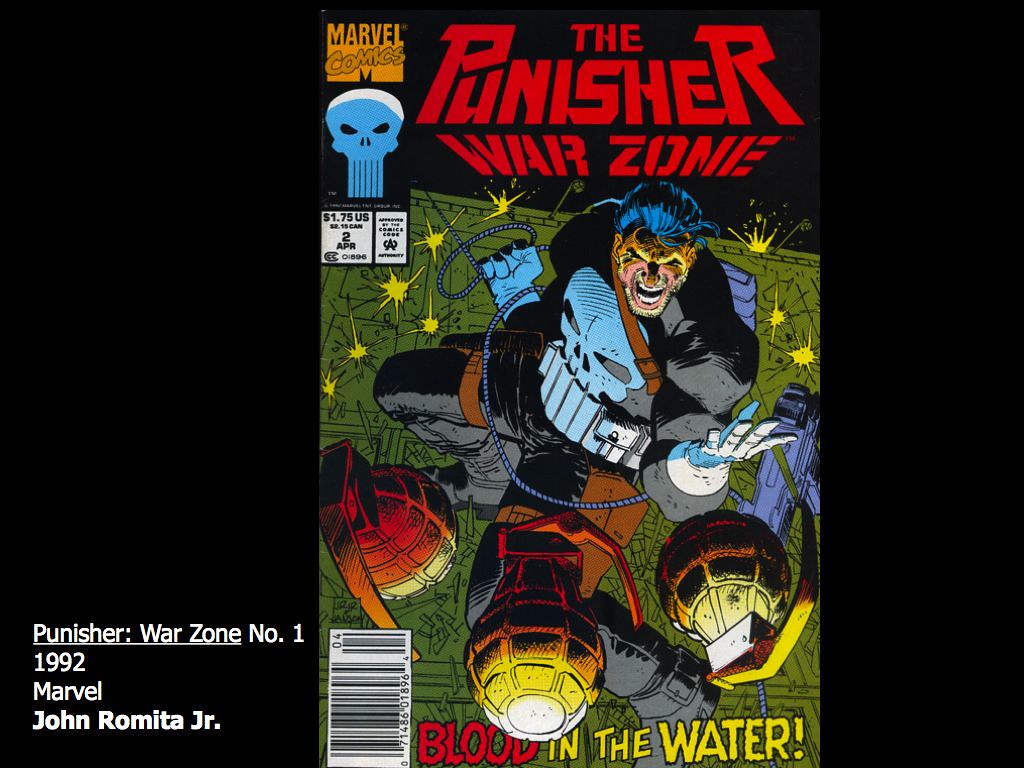The comic book cover features "The Punisher: Warzone" in bold red text at the top, with the subtitle "Blood in the Water" underneath— "Blood" in red and "In the Water" in yellow. The left side of the cover has a vertical black border containing the text "Punisher Warzone, Number One, 1992, Marvel, John Romita Jr." in white. The top left corner of the cover showcases "Marvel Comics" in orange text, accompanied by a white and blue skull motif missing its bottom jaw.

Dominating the center of the cover, The Punisher is depicted wearing a tight black suit with a large, elongated blue skull emblem on the chest. He sports white gloves and a serious expression as he appears to be in mid-action—either punching or flying—while throwing three large fragmentation grenades behind him, which are shown prominently in the foreground. The scene is marked by dynamic star-like symbols indicating bullet fire, adding to the intense, action-packed atmosphere of the image.